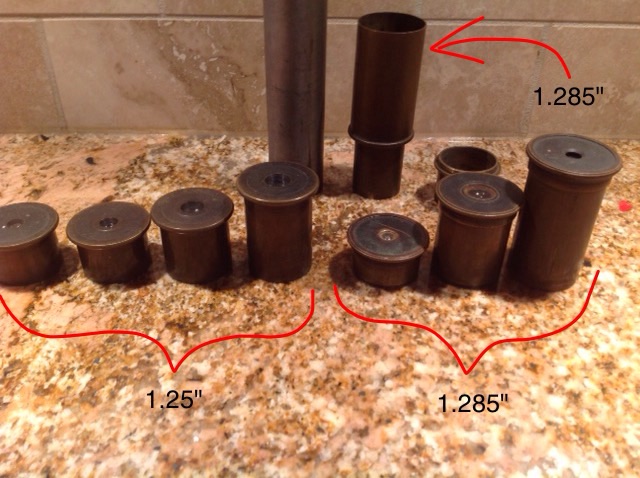This is an indoor, natural light, full-color photograph featuring an assortment of metallic, brass or copper-colored cylindrical pieces resembling shell casings with flat, flared tops and central screw holes. The image is set on a brown, flecked granite countertop with a light brown tiled wall in the background, suggesting a kitchen or bathroom setting. 

The metallic pieces are arranged in distinct groupings. To the left, four pieces are lined up and gradually increase in height; these are labeled with a red parenthesis that notes their measurement as 1.25 inches. In the center, two pieces are positioned behind the front row, each indicated by a red arrow labeled 1.285 inches. On the right, three additional pieces, also increasing in height from left to right, are marked with another red parenthesis indicating 1.285 inches. The meticulous arrangement and precise measurements highlight the varying heights of these small metal components.